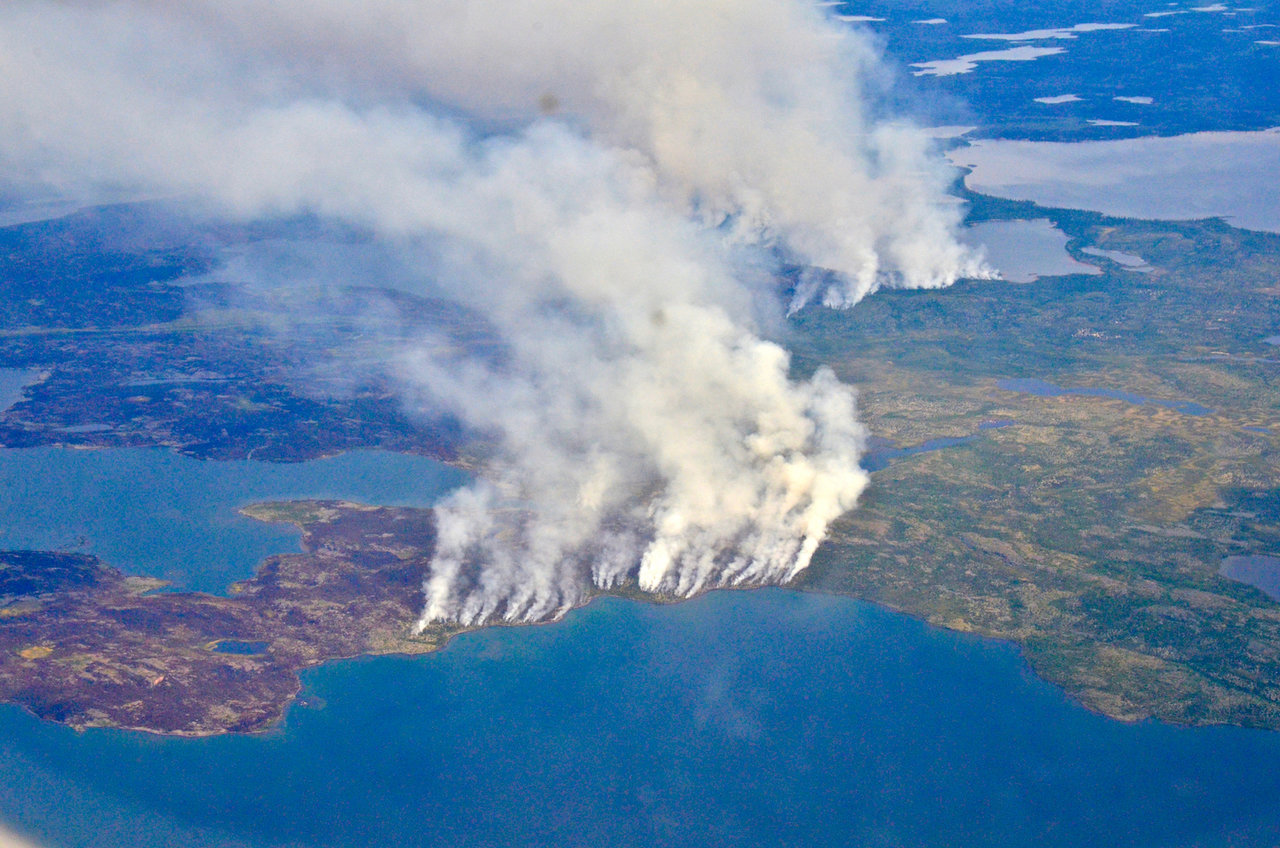This aerial photograph captures a dramatic scene of a landscape engulfed in multiple wildfires. Taken from a high altitude, likely from an airplane or helicopter, the image shows a large island surrounded by deep blue ocean waters. The central focus of the image is the extensive plumes of white and light gray smoke billowing up from various parts of the land, particularly along the coastline. 

The landmass itself is varied in color, featuring dark brown, light brown, green, and yellow patches, indicating diverse terrain and vegetation possibly already affected by the fires. The northwest section of the island reveals another intense plume of smoke, suggesting another active wildfire. The smoke from these fires rises in substantial spirals, merging into a thick, grayish cloud cover obscuring parts of the sky.

Despite the height from which this image is taken, some details like the contrast between the dark, burned areas and remaining green vegetation are visible. The image offers a stark contrast between the serene blue of the surrounding ocean and the chaotic, smoke-filled landscape of the island, strongly implying the severity of the wildfires. The overall composition of the photograph illustrates a significant environmental event, with widespread smoke impacting several miles of shoreline and further inland areas.